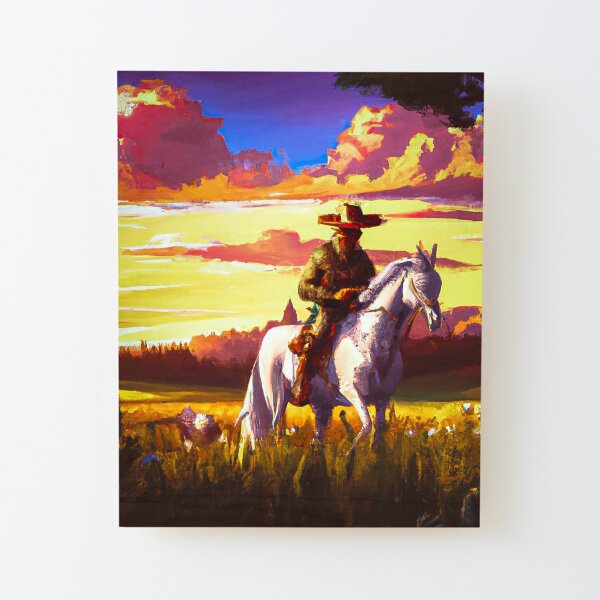In this vivid painting, likely available for purchase on a canvas website, a scene unfolds of a cowboy—or possibly a bandito—atop a striking white horse. The cowboy is dressed in full traditional attire, including a brown jacket, brown pants, brownish-red boots, and chaps. His face is partially obscured by a red bandana, adding an air of mystery. He wears a distinctive hat, possibly a sombrero, setting him apart from the typical cowboy image. 

The white horse is equally adorned, featuring a saddle and a white bandana, with a long, flowing mane and tail. Both horse and rider appear to be steadily moving through a tall, green grassy field dotted with white flowers.

The backdrop showcases a dynamic sky where day transitions to night: the upper expanse is a lighter blue, deepening into indigo, and fading into hues of yellow, pink, purple, and orange as the sun sets. Clouds add dramatic contrast, some tinged with purples and oranges, while one darker, tree-like silhouette stands prominently. Further enhancing the scene's depth are a row of gentle hills and a castle peeking through a cloud formation, creating a picturesque, almost storybook quality to the imagery. The entire composition is bathed in the warm, golden light of the setting sun, which casts a gentle glow on both the horse and the cowboy, enriching the scene with a sense of timeless adventure.